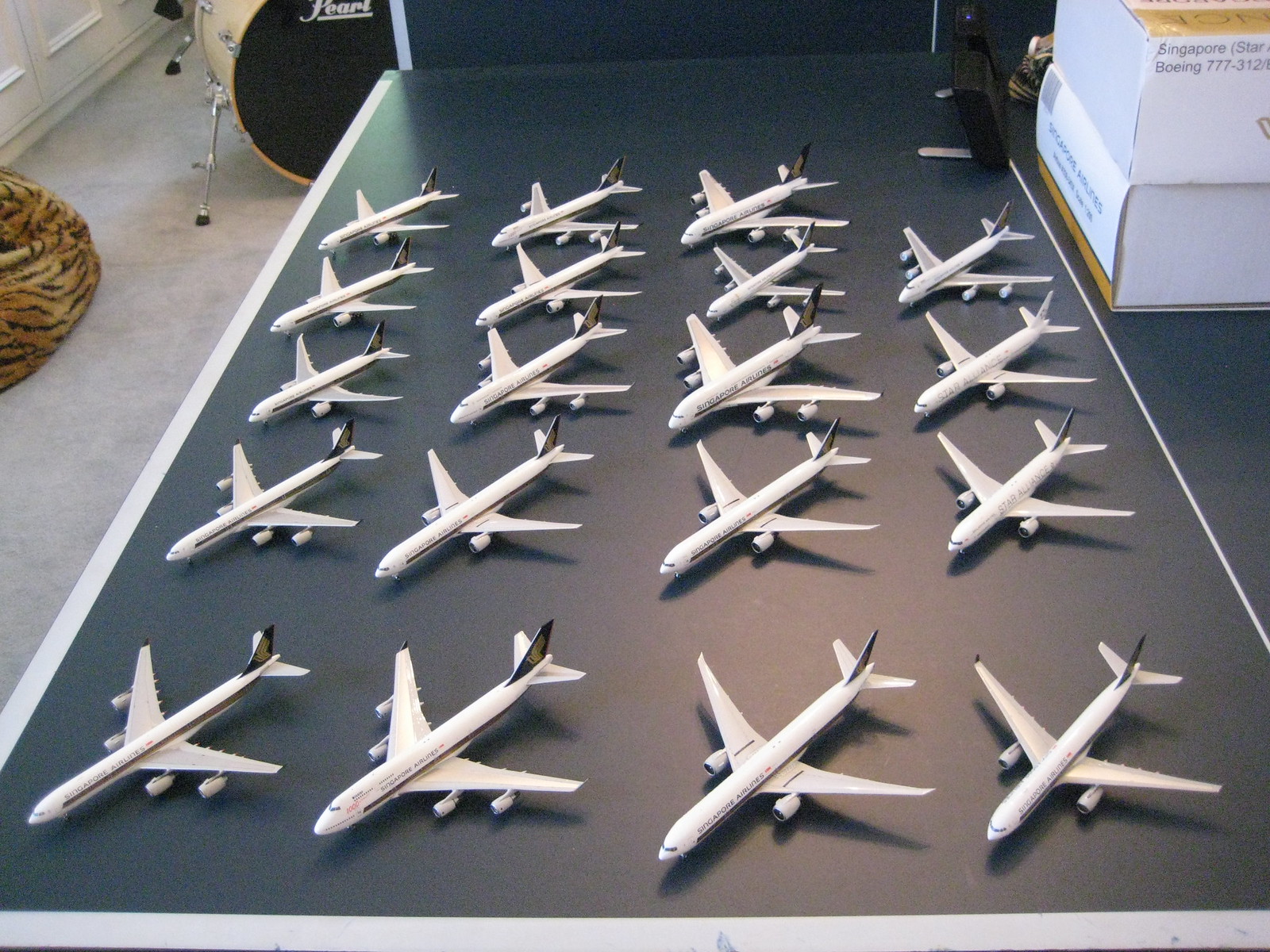The image features a detailed display of 19 small-scale model airplanes meticulously arranged on one half of a navy blue ping pong table with white lines. The airplanes, primarily white with British Airways insignia, are organized in rows—four rows of four and one row of three— all facing the same direction. On the right side of the table lies a box labeled "Singapore" and "Boeing 777," potentially indicating the model type of some displayed planes. The surrounding area provides additional context: a gray cement floor, a small piece of a drum kit in the top left corner, and a tiger print bean bag near the right edge. The setting appears to be a garage or storage room, further hinted by the visible carpet and wall in the background.